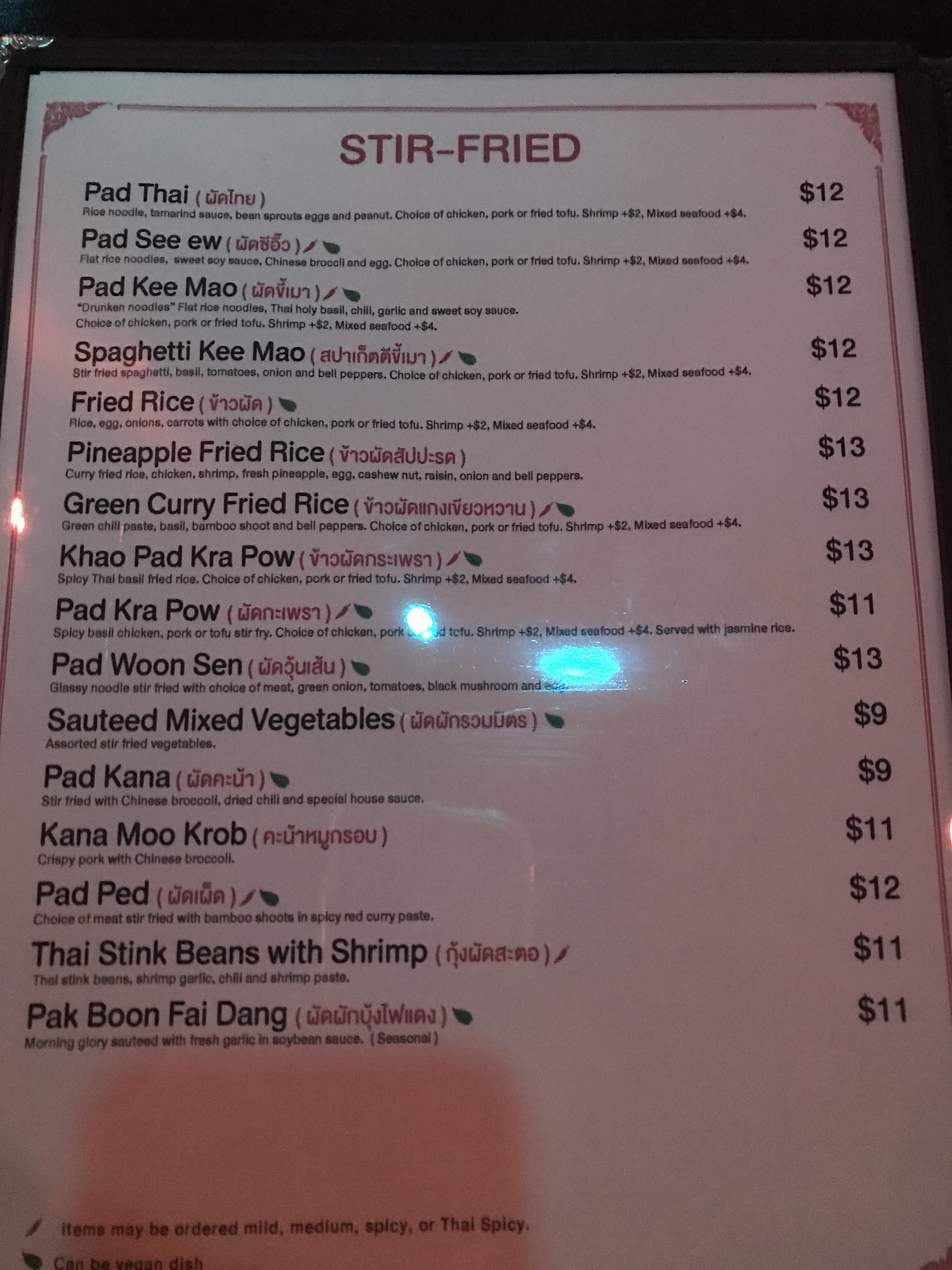The menu, possibly from a Thai restaurant, features a collection of dishes under the header "Stir Fried" prominently displayed in large red letters at the top of a white sheet of paper. The menu appears to be either laminated or enclosed in a transparent plastic folder. The paper itself has a distinct red border. 

Each dish is listed with its name in black text, accompanied by a translation in smaller red text, likely in Thai. The dishes include Pad Thai, Pad Siu, Pad Kemau, Spaghetti Kemau, Fried Rice, Pineapple Fried Rice, Green Curry Fried Rice, Khao Pad Krapow, Pad Krapow, Pad Woon Sen, Sautéed Mixed Vegetables, Pad Khana, Khanam Krob, Pad Ped, Thai Stink Beans with Shrimp, and Pak Boon Fai Dang. Detailed ingredients for each dish are printed below in smaller text. 

The prices for these meals range from $9 to $13, with each price clearly marked in dollars next to the respective dish.